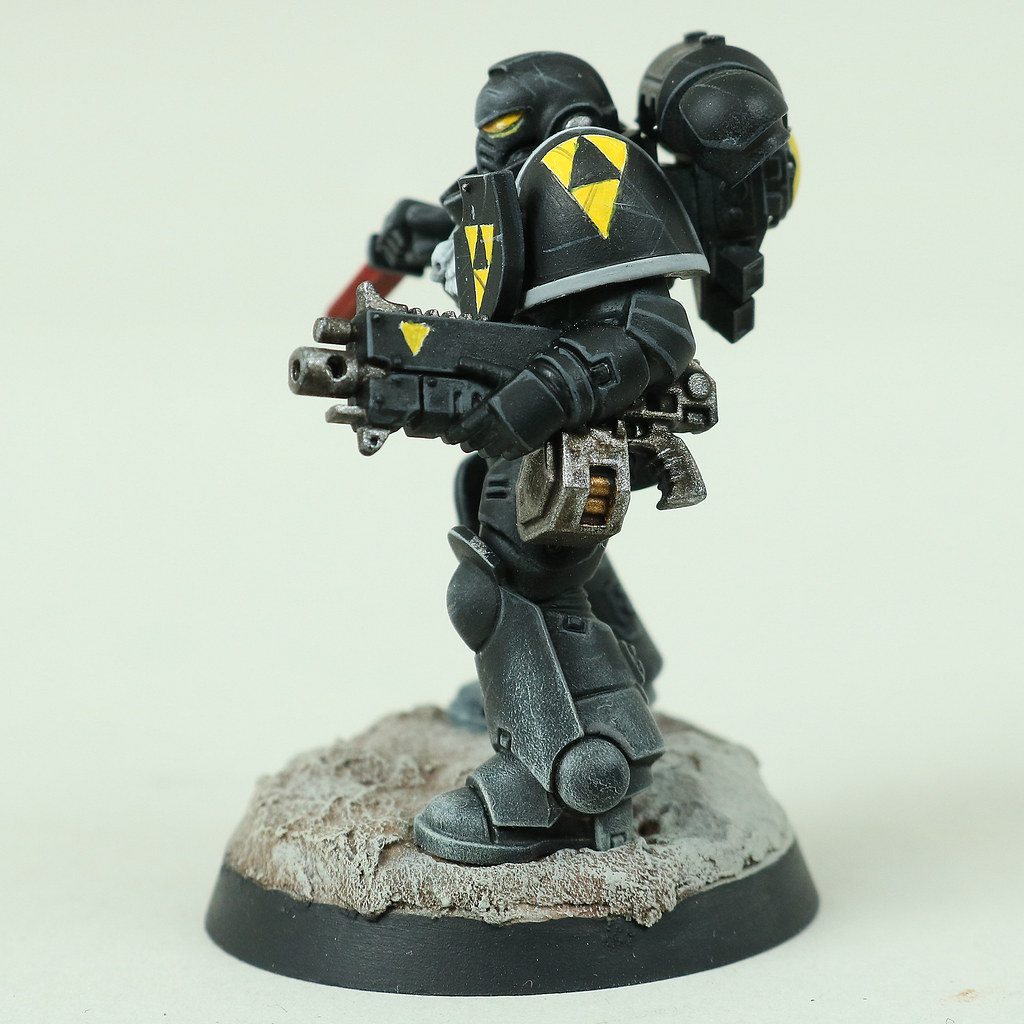The image depicts a detailed, small painted figurine of a heavily armored, bipedal humanoid space marine standing on a sandy or dirt-colored platform with a black base. The figurine, facing left, is adorned in grey metallic armor and features large shoulder pads, a small shield on its chest, and a biohazard-like symbol—black triangles inside yellow triangles—on its shoulders. The space marine has yellow eyes and wields a large metallic-looking grenade launcher in its left hand and an orange-bladed knife in its right. Additionally, another weapon can be seen strapped to the figurine's back. The entire scene is set against a solid white surface and background, giving prominence to the detailed and intricate work of the figurine.